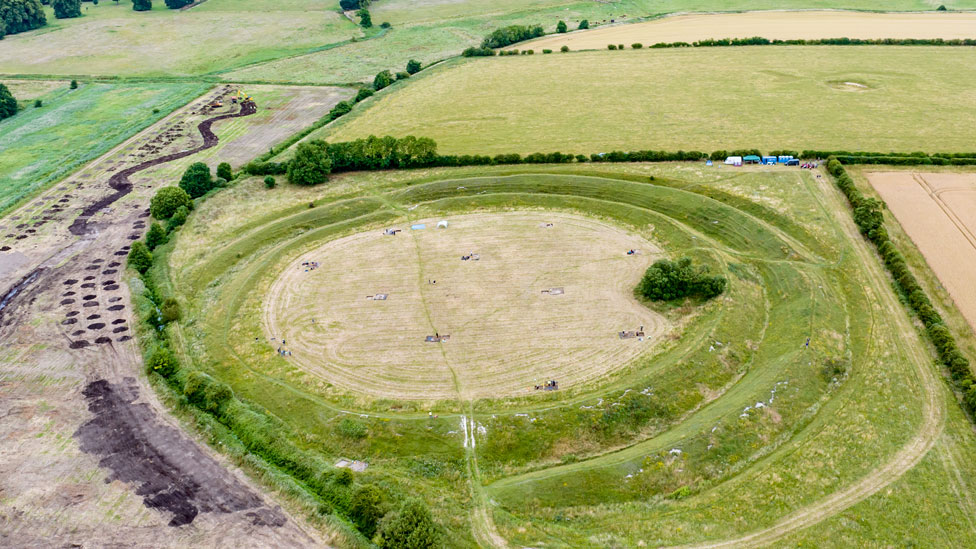This aerial photograph captures a detailed view of an open and expansive agricultural field. Dominating the scene is a striking circular area in the foreground, mowed closer than the surrounding land, resulting in a distinctive golden-green hue contrasted against the deeper green of the adjacent fields. This circular pattern suggests recent activity, possibly for tilling, or it could have been prepared for an event, given its worn appearance and visible tire tracks weaving in and out. Within this circle, a central beige area contains boxes or equipment, hinting at ongoing agricultural operations. To the right, small clusters of trees and possible food trucks are present, indicating some human congregation or perhaps preparation for a festival.

The landscape is segmented into four or five rectangular plots, each bordered by tree lines, contributing to an orderly yet varied patchwork of textures and colors. These plots feature different states of cultivation, with some showing bare patches and others appearing sandy or dotted with holes, adding to the complexity of the terrain. The photograph also reveals subtle elevation changes, with the land contouring gently upwards and downwards, suggesting a man-made influence over the natural landscape. Tucked into corners and edges of these plots are hints of housing or additional equipment, further emphasizing the multifunctional use of this agricultural space.